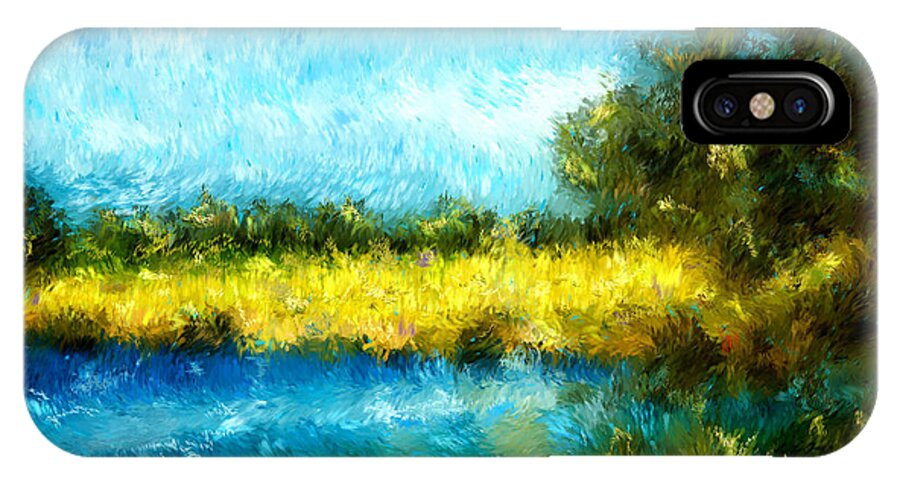The photograph features the back of a cell phone, specifically standing on its long edge, emphasizing its decorative case. The case showcases a pastel artwork reminiscent of Cézanne or Van Gogh's style, predominantly nature-themed. The scene painted on the case includes a sky blue top with subtle white highlights, transitioning into a meadow of greenish-tan hues beneath it. Along the top edge of the meadow, green bushes are depicted, likely due to their height. To the right side of the painting, larger bushes or trees create a denser overgrowth. At the very bottom, a darker blue area suggests the presence of water, reflecting the sky above. The camera lenses, characteristic of an iPhone X, are located in a black oval on the upper right corner of the phone. The case is vividly colorful, featuring greens, blues, and golden hues, and captures a visually stunning, abstract nature scene, with swirly lines and detailed artwork that might be more discernible from a distance.